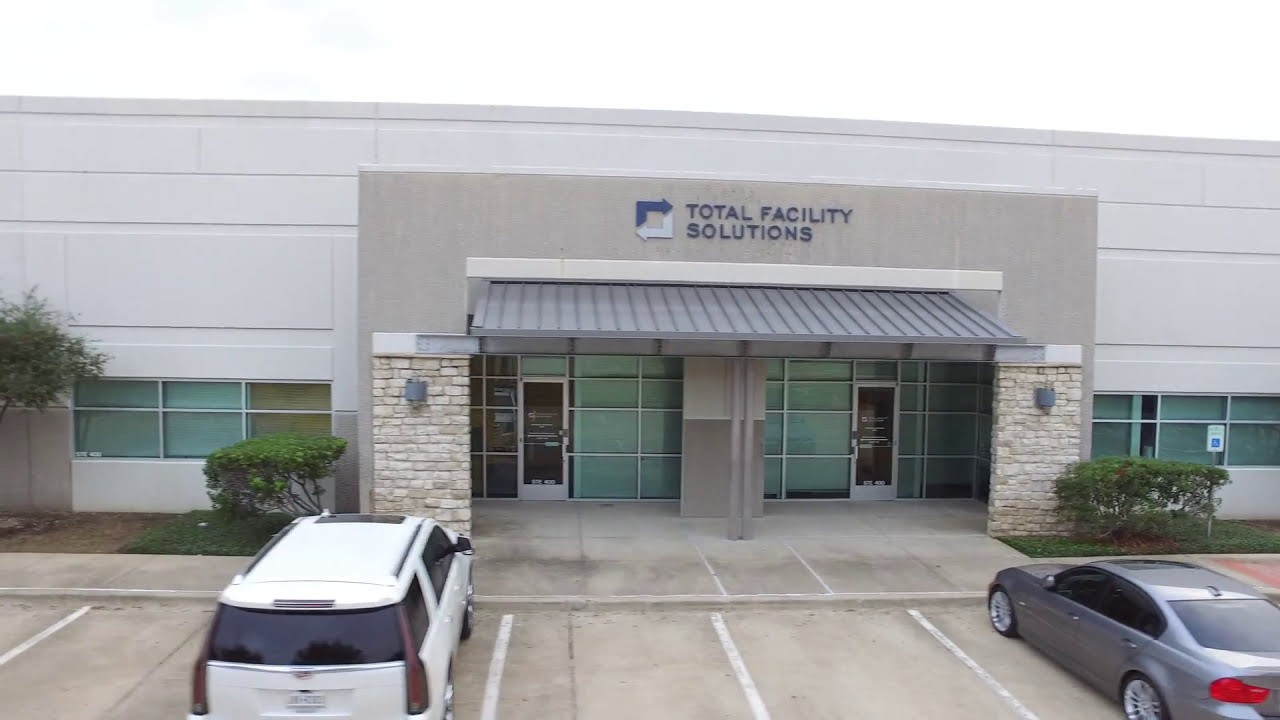The image showcases the exterior of a two-story, light gray concrete building with the name "Total Facility Solutions" prominently displayed in blue capital letters on a sign above the double doors. The logo, consisting of two arrows forming a square, is also visible on the sign. This structure has the characteristic appearance of a warehouse or manufacturing plant.

In front of the building is a parking lot with a few green shrubs flanking the entrance. There are two vehicles parked close to the entrance: a white SUV to the left and a silver sedan to the right. Besides these two occupied spots, there are approximately four or five additional empty parking spaces, including a visible handicapped parking space near the gray sedan.

The building facade features stone columns and multiple windows with shades, as well as two lights. Each of the entrance doors bears white writing. The overall scene is devoid of people, and the sky overhead is gray, adding a subdued quality to the environment.